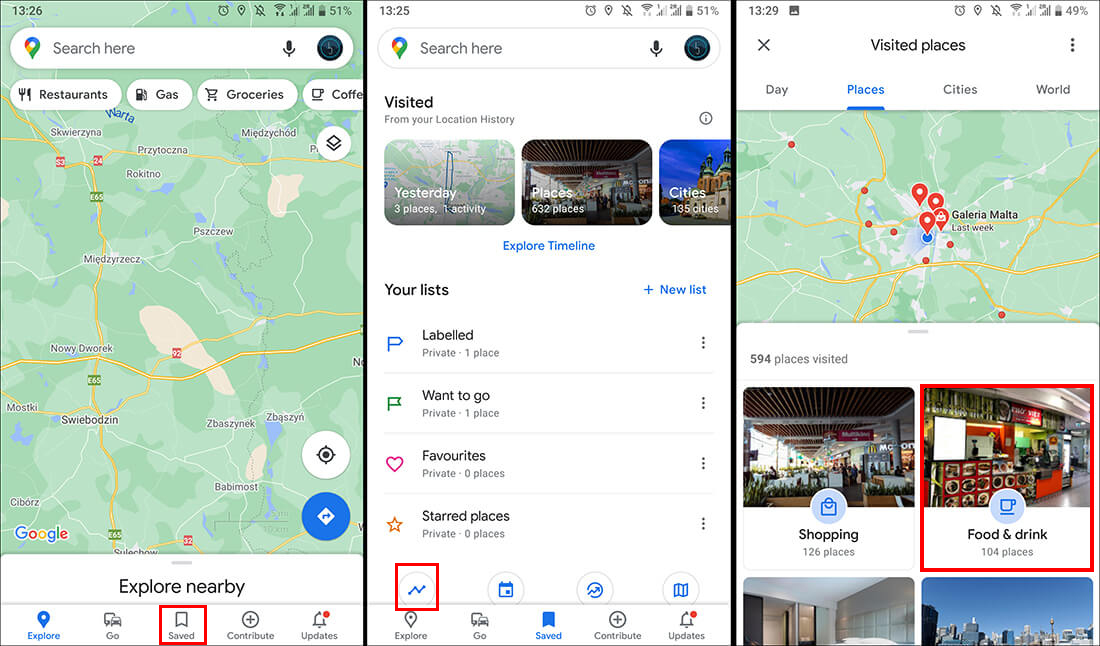The image displays three consecutive screenshots from Google Maps, each providing a different set of details regarding a user's recent activities and saved places:

1. **First Screenshot (13:26)**:
   - Detailed Google Maps view with the multicolored location pin and “Search here” text in a white oval at the top.
   - The app displays options such as "Explore nearby," "Restaurants," "Gas," "Groceries," "Coffee," and a layers symbol.
   - The "Save" option is highlighted with a red box, indicating current selection.
   - The location language suggests the map might be covering an area in Sweden, Denmark, Russia, or Germany, with text containing more z's than typical English words.

2. **Second Screenshot (13:25)**:
   - The screen shows the user's location history with a map of visited places indicated by lines.
   - The timestamp suggests it captures data from the previous day.
   - It summarizes the user’s travel log: "632 places visited" and "135 cities".
   - Options include "Explore timeline," "Your lists," and "Add a new list."
   - Lists are categorized as "Private," denoted by a blue 'P' icon, "Want to go" with a green sign, "Favorites" with a heart, and "Starred places" starring zero entries.

3. **Third Screenshot (13:29)**:
   - Featuring "Visited places" with categories: "Day," "Places," "Cities," and "World," with "Places" being selected.
   - The entry for "Galleria Malta" is noted as visited last week.
   - There are four location pointers indicating various places visited around Galleria Malta, specifically to the southwest, though distances aren't precisely readable.
   - Overall visitation stats include "594 places visited," "126 shopping places," and "104 food and drink places."
   - The current selection around "Food and Drink" is marked by a red box, indicating the user’s search interest in restaurants or eateries at the moment.

Overall, the screenshots offer a comprehensive overview of recent travel activity and places the user is interested in, oriented around both saved searches and historical visit data.